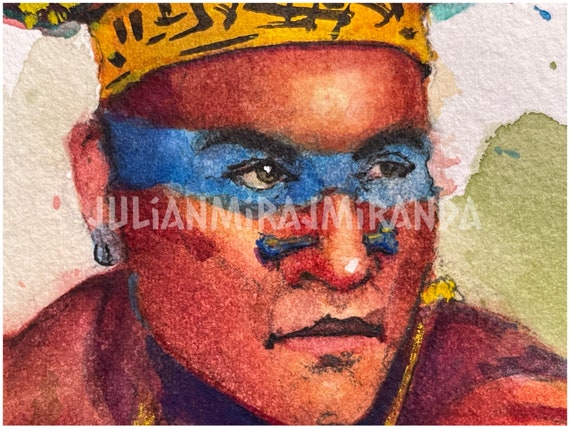The image is a detailed watercolor painting focusing on the face of an indigenous man. The name "Julian Mira, E. Miranda" appears as a watermark in the center of the painting. The man's skin tone is rendered in a vivid ruby red, with a striking blue streak of face paint extending across his eyes from ear to ear, resembling a mask. The blue paint covers his eyebrows and eyes, giving him an adorned appearance. His nose is pierced at the mid-bridge with a blue adornment, possibly resembling a bone earring or nose ring. The stern expression on his face captures attention, with his gaze directed to his left. A yellow headband with black lettering, likely in an unknown language, encircles his head. The painting showcases a vibrant palette, including reds, blues, whites, and greens, adding depth and richness to the artwork. Only the man's shoulders are visible, suggesting he is wearing a coat, and the overall composition emphasizes the intricate facial details and ceremonial adornments.